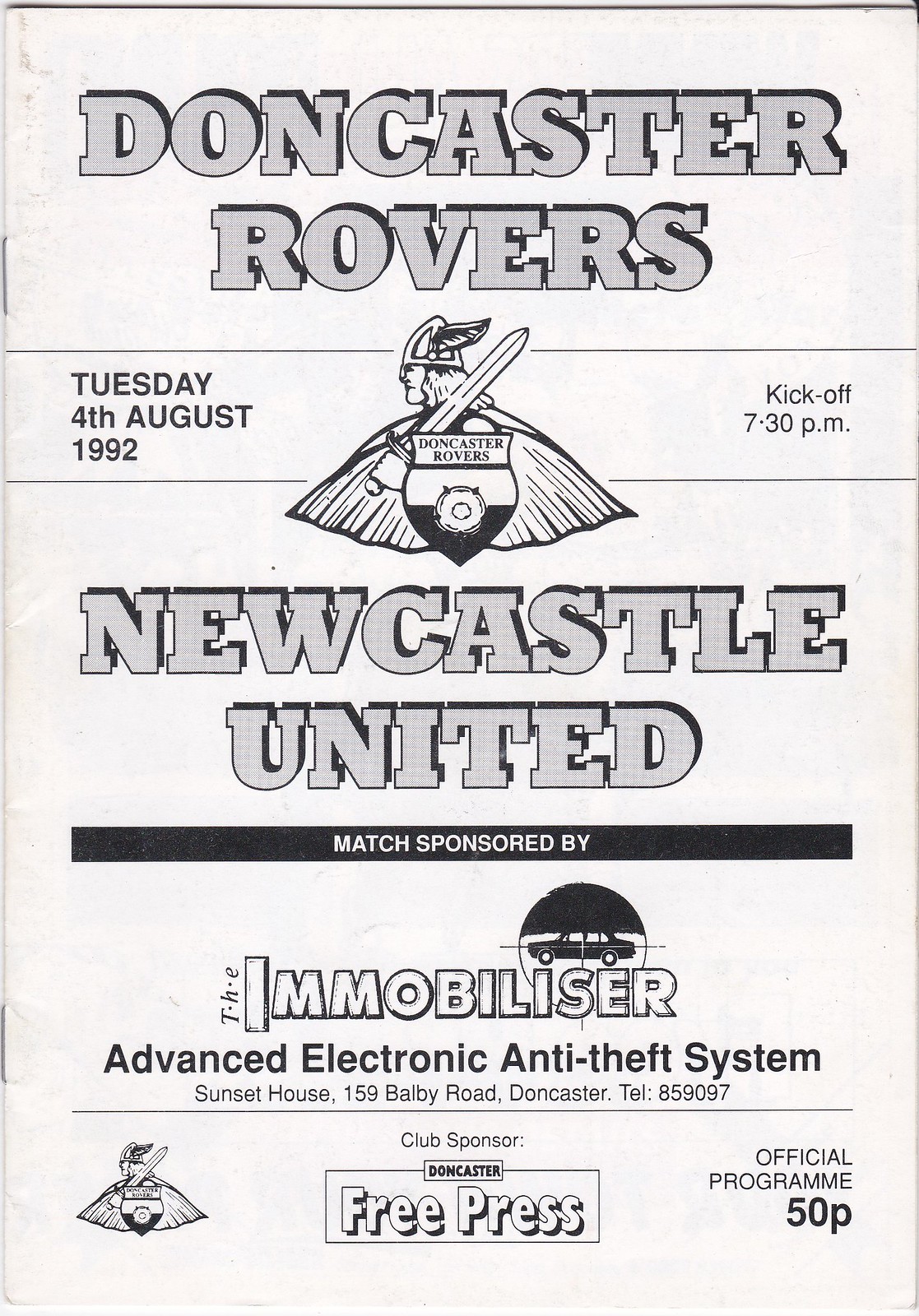This is a detailed black-and-white image of the front page of a program for a soccer match. At the top, "Doncaster Rovers" is prominently displayed in gray letters against a white background, accompanied by the Doncaster Rovers' symbol. To the left, the date "Tuesday, 4th August, 1992" is listed, while the kickoff time, "7.30 p.m.," is noted on the right. Below, "Newcastle United" is written in large gray letters. Further down, the match is noted to be sponsored by "Immobilizer," which is emphasized in big white letters. Underneath the sponsor's name, it says in black, "Advanced Electronic Anti-Theft System," followed by an address: "Sunset House, 159 Dalby Road, Doncaster." At the very bottom of the page, "Club Sponsor, Doncaster Free Press" is mentioned. On the left corner of the page, the Doncaster Rovers' symbol reappears, and on the right, it states, "Official Program, 50P." Additionally, a car logo is visible in front of the "Immobilizer" text, reinforcing the automotive theme of the sponsor.